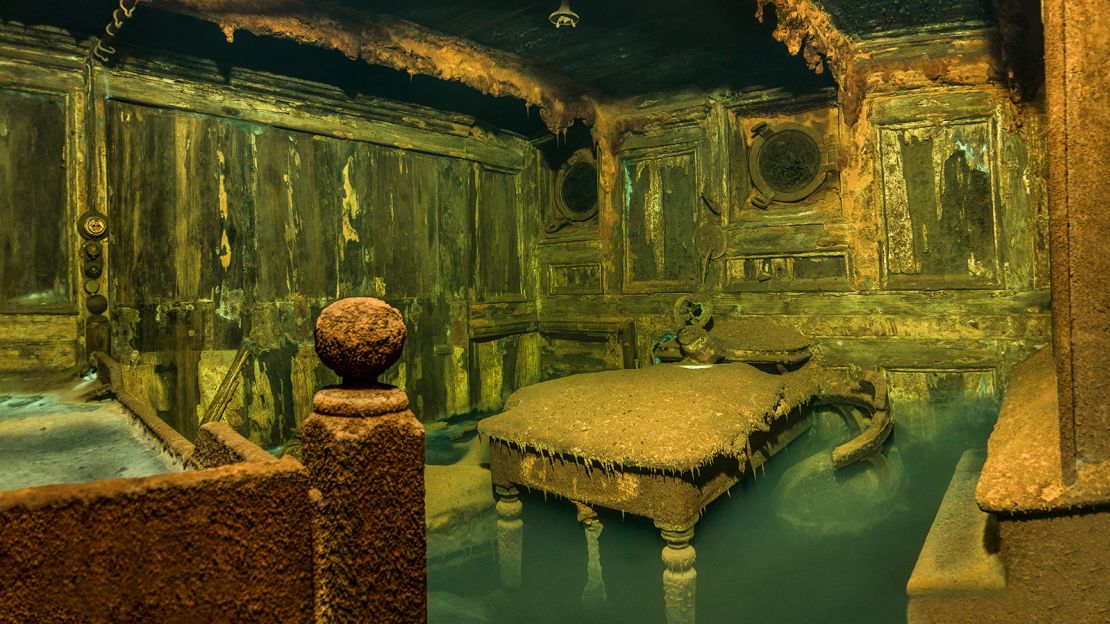The image displays a horizontally rectangular photograph capturing the interior of a decayed, waterlogged room, suggestive of a shipwreck submerged for a prolonged time. The room is small and rectangular, with muted, earthy tones—predominantly brown and green—dominating the scene. The walls are streaked with light brown and green, showing severe water damage and rot, exuding a feeling of abandonment and antique age.

Prominently, a bed is positioned against the back wall, its wooden or metal frame rusted and crusty, with a mattress that has deteriorated into a yellowish hue. Beneath and surrounding the bed, murky green water partially submerges the furniture, reflecting light from unidentified sources above. A further detail includes old, rotted-away paintings hanging on the moisture-ravaged walls, barely identifiable as frames.

Additional room features include a brown crusty banister on the lower left and small porthole windows on the back wall, hinting at the room's nautical origins. The setting is accentuated by the presence of barnacle-like growths on the ceiling and various hanging, deteriorated elements, intensifying the overall impression of an underwater relic steeped in history and decay.